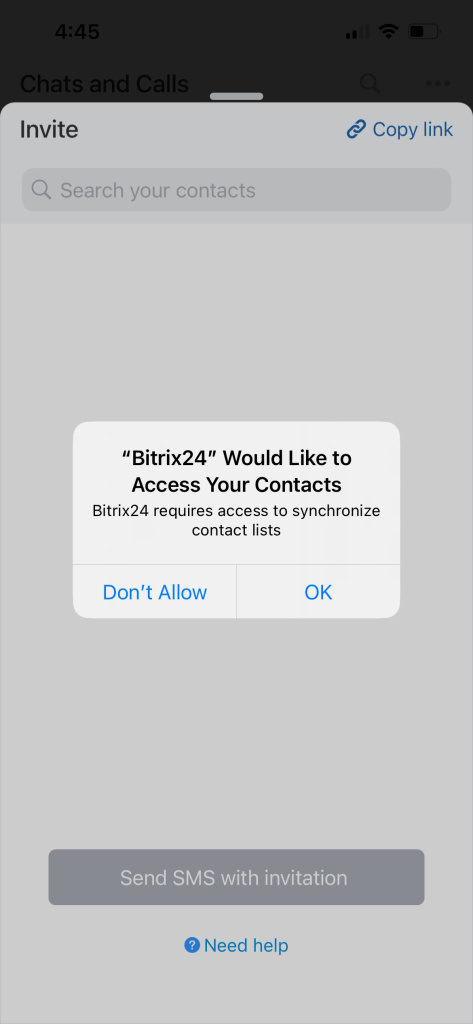The image is a screenshot from a cell phone displaying a request for access in a pop-up notification. The background of the screen is originally white, but due to the pop-up, an opaque light gray overlay makes the background appear gray. At the top of the screen, there is a black bar. Underneath this bar, the visible but partially obscured background contains the word "Invite" in the top left corner and "Copy Link" in the top right corner. Below these options is a search bar labeled "Search your contacts."

The central focus of the image is a white, landscape-oriented rectangular pop-up. This pop-up displays a message in quotation marks that reads, "Bittrex24 would like to access your contacts." Following this, the pop-up explains, "Bittrex24 requires access to synchronize contact lists." Below the text, there are two buttons: "Don't Allow" and "OK," both written in blue against a white background.

Beneath the pop-up, the remaining visible part of the background shows a dark gray button labeled "Send SMS with Invitation." At the very bottom of the screen, a blue circle featuring a question mark is center-justified, accompanied by the text "Need help."

The detailed composition of the screenshot captures both the interface elements and the specific permissions request, providing a comprehensive overview of the display.